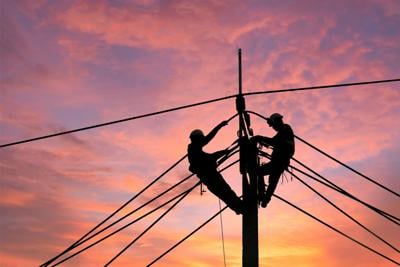In this artistic full-color photograph taken outdoors at either sunrise or sunset, the vibrant sky serves as the dramatic backdrop for two silhouetted linemen working on a power line. The sky is a canvas of vivid hues, transitioning from yellow, orange, and red at the horizon, where the sun is rising or setting, up to sporadic pink and purple clouds with patches of blue. From the bottom, slightly to the right of the center, a utility pole ascends, nearly reaching the middle of the image. Two men, secured with belts and wearing helmets, are positioned on either side of the pole, each holding onto the wires. The scene captures the intricate web of electrical wires stretching both vertically towards the ground and horizontally above the men's heads, accentuating the contrast between their dark silhouettes and the illuminated sky.